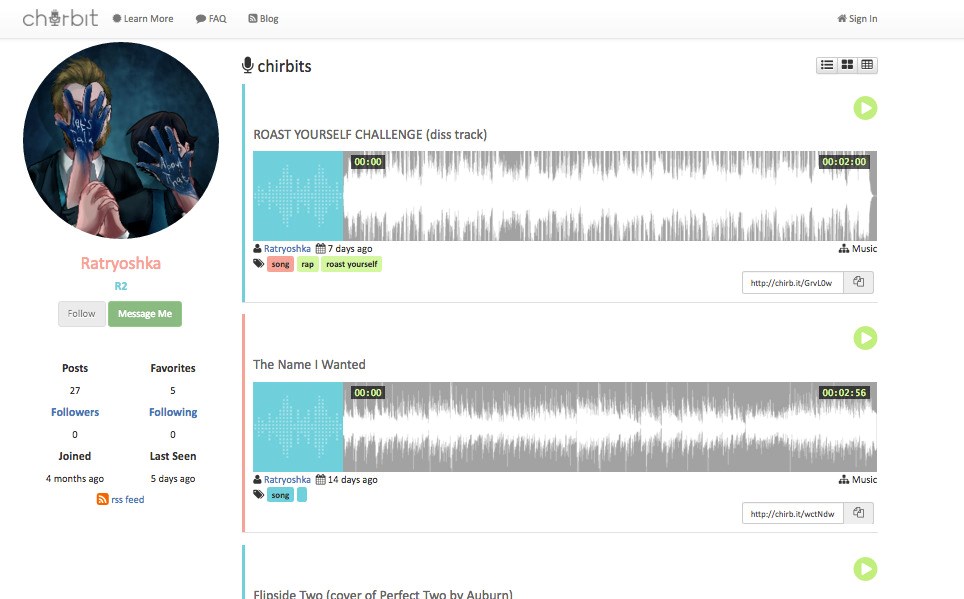The top of the image displays a header labeled "CHRBIT," with an unidentified icon situated between the letters "H" and "R." Adjacent to this header are navigation links labeled "Learn More," "FAQ," "Blog," and "Sign In."

Beneath the header, on the left side, there is an oval-shaped image featuring an illustration. The illustration depicts two individuals, one of whom is dressed in a suit with their hands covering their face, smeared with blue paint. Below this illustration is the text "Rastriyashka R2." Accompanying this are two buttons: a gray "Follow" button and a green "Message Me" button.

Further down, there is a user information section listing the following details:
- Posts: 27
- Favorites: 5
- Followers: 0
- Following: 0
- Joined: Four months ago
- Last seen: Five days ago

On the right side of the image, there are two audio waveforms representing sound files. The first file is titled "Roast Yourself Challenge Diss Track" with a duration of two minutes. The second file is titled "The Name I Wanted" and is two minutes and 56 seconds long.